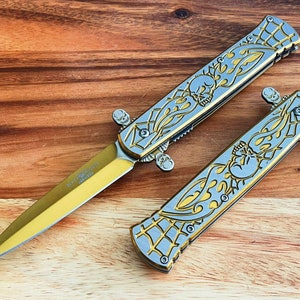This image features a detailed knife set against a wooden table that transitions from dark at the top to lighter towards the bottom. The primary knife, possibly a switchblade, stands out with a silverish-blue handle and a striking yellow-gold blade adorned with etched skull designs. These skulls, appearing both large and small, seem to have an angry expression and are accompanied by intricate spiderweb engravings. The smaller skulls extend from the sides of the blade, adding to its menacing aesthetic. In the background, a second knife, partially visible, mirrors the same design elements—skull and spiderweb motifs etched in silver with a yellow-gold backing—completing the hauntingly detailed composition.